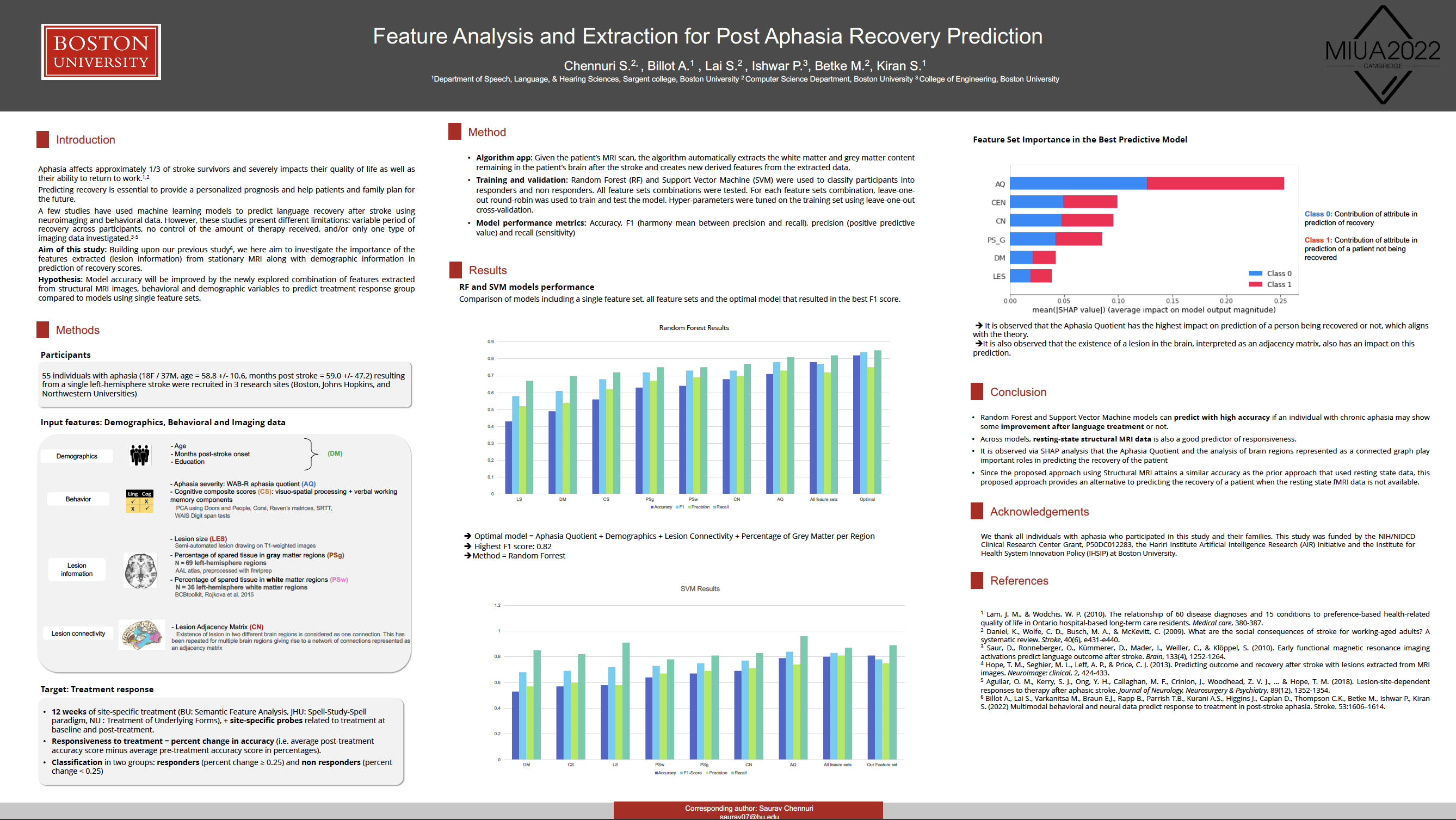This image is a detailed screenshot of a webpage from Boston University, as indicated by the logo on the top left. The central theme of the page, titled "Feature Analysis and Extraction for Post-Aphasia Recovery Prediction," is presented in white lettering against a gray backdrop at the top. Below the title, the content is divided into multiple sections with headings in red, such as "Introduction," "Methods," "Results," "Conclusion," "Acknowledgment," and "References." 

The visual elements include a variety of bar charts and line graphs. At the top, several vertical bar charts use shades of blue and green to distinguish different data points, while on the right side, there are horizontal bar charts that employ blues and reds. Additionally, a section on the left features illustrations that include stick figures, check marks and X's, and images of a human brain, seemingly to explain the chart data. Despite the densely packed paragraphs of text, the information appears too small to read in detail. MUA 2022 is also noted on the right side of the top banner, adding context to the project's scope or event.